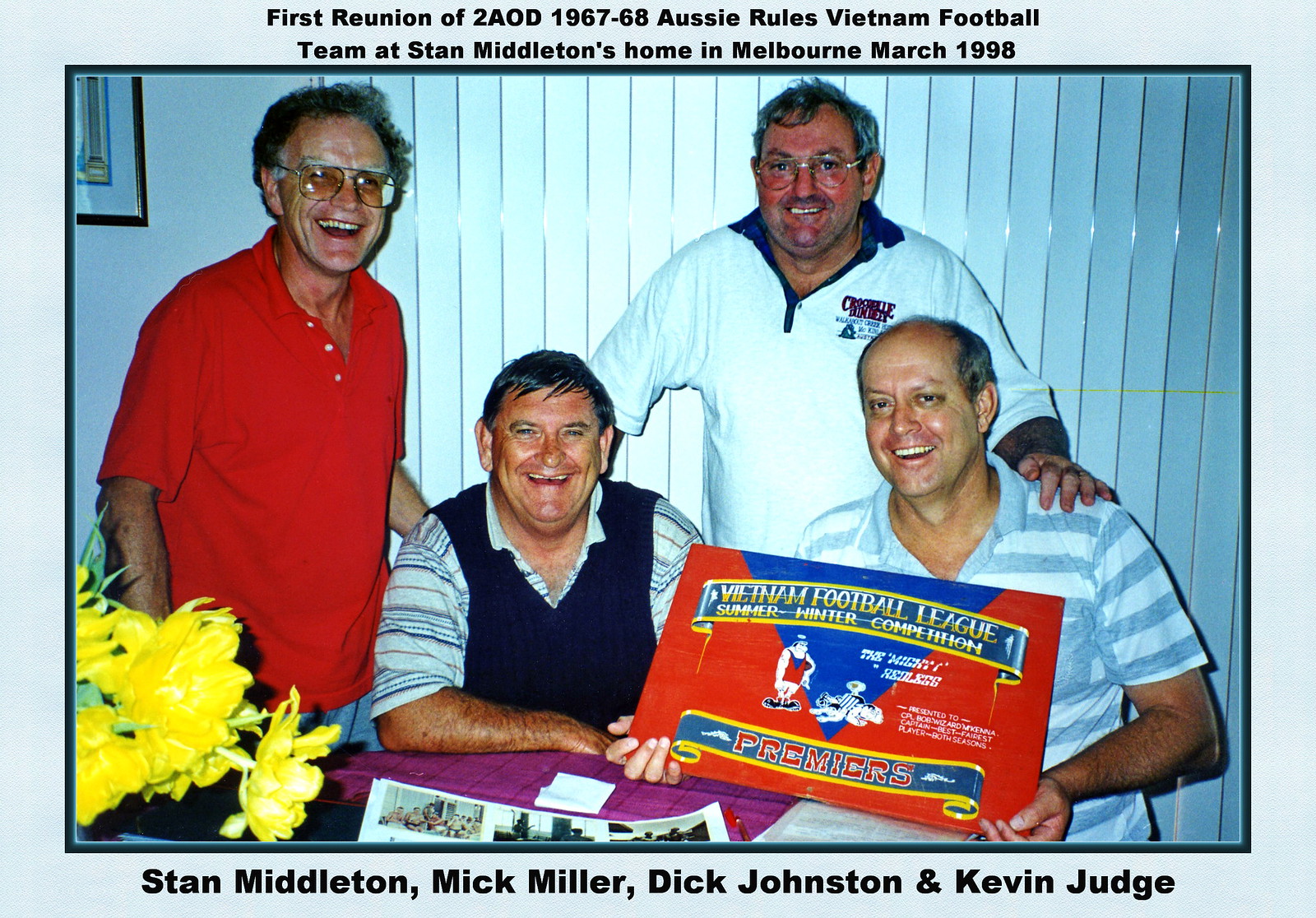A group photo captures four older gentlemen, who are identified from left to right as Stan Middleton, Mick Miller, Dick Johnston, and Kevin Judge. They are presumably sitting at a kitchen table inside Stan Middleton's home in Melbourne during the First Reunion of the 2AOD 1967-68 Aussie Rules Vietnam Football Team, which took place in March 1998. Stan Middleton, on the far left, is standing and wearing a short-sleeved red polo shirt and thick glasses, smiling openly at the camera. Seated next to him is Mick Miller in a blue vest over a white and blue striped short-sleeved shirt, also smiling directly at the camera. Behind Mick Miller and slightly to the right stands Dick Johnston, wearing a white shirt with a blue collar and glasses, with his hand resting on the shoulder of Kevin Judge. Kevin, seated at the far right, holds up a large piece of red cardboard that reads "Vietnam Football League Summer Winter Competition Premieres" and features cartoon characters in soccer uniforms. The image is bordered by a light bluish-gray frame with a header stating, "First Reunion of 2AOD 1967-68 Aussie Rules Vietnam Football Team at Stan Middleton's Home in Melbourne, March 1998," and a footer labeling each person in the photo.